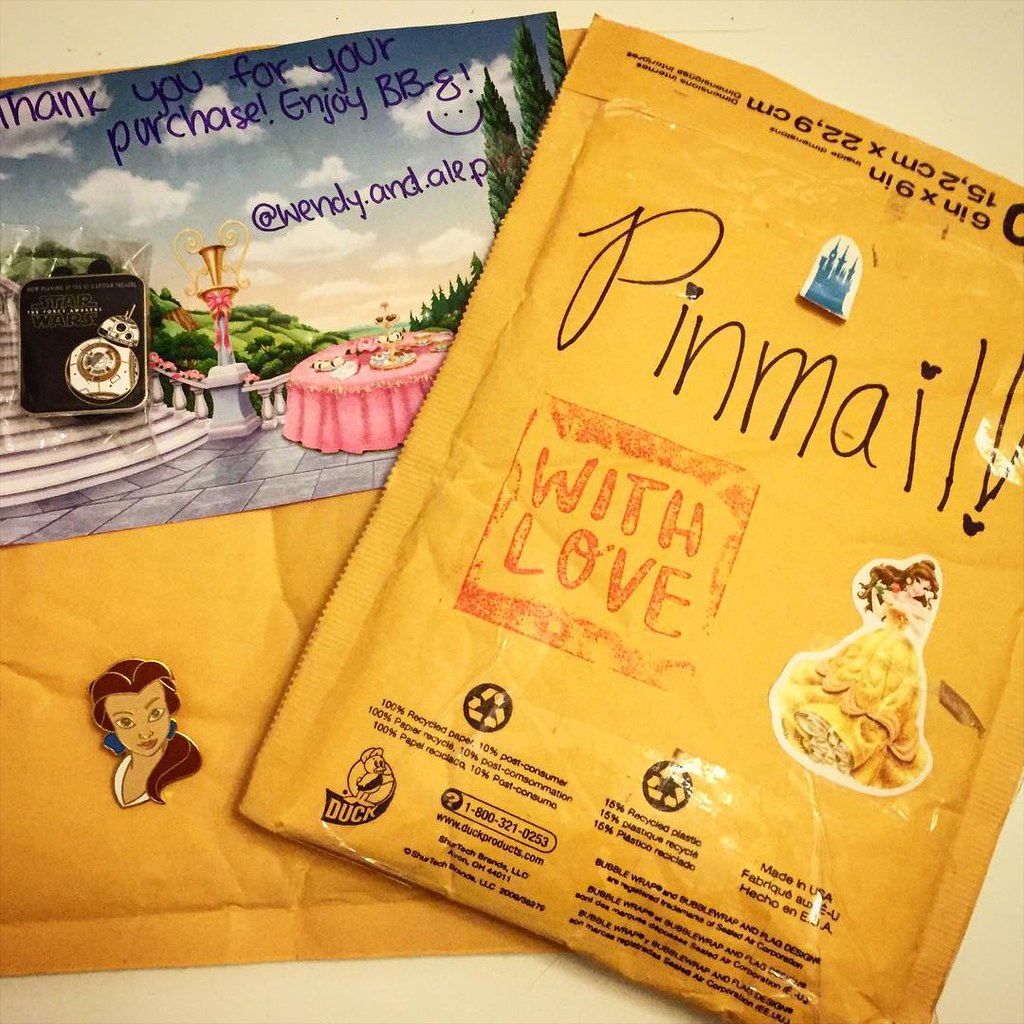The square image showcases a pile of mail on an off-white, yellowish surface visible at the edges. The mail consists of two large, overlapping yellow manila envelopes. The top envelope is a tall rectangle, tilted diagonally clockwise, with its right corner cut off by the edge of the image. Written in black marker on this envelope are the words "Pin Mail!" next to a red stamp that reads "With Love." To the right of the stamp is a sticker of Belle from Beauty and the Beast, wearing a yellow-gold dress and with long brown hair. The bottom envelope lies more straight, partially covered by a printed piece of paper that says, "Thank you for your purchase, enjoy BB-8!" with a smiley face. The paper also contains animated images of a staircase leading to a castle, a table with food, mountains, and trees in the background. Another Belle sticker sits at the bottom of this envelope. Additionally, there's a square pin with rounded corners featuring BB-8 on top of the bottom envelope. This highly detailed arrangement suggests a personalized, decorated mailing experience.